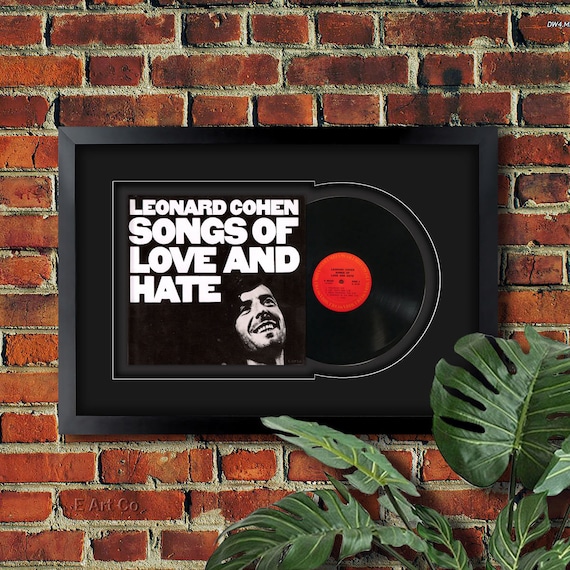This image features a commemorative plaque celebrating the release of Leonard Cohen's album "Songs of Love and Hate." The plaque is presented within a rectangular black frame and set against a red and brown face brick wall. The album cover, showcasing white lettering that boldly states "Leonard Cohen" and below it "Songs of Love and Hate," also includes a black-and-white picture of Leonard Cohen on the bottom right. Intriguingly, the vinyl record is partially pulled out of its sleeve, with about three-quarters of it exposed, revealing a red sticker in the middle of the disc. In front of the framed album, there is a greenhouse plant in a pot, positioned on the floor, its foliage partially obscuring the bottom of the frame.